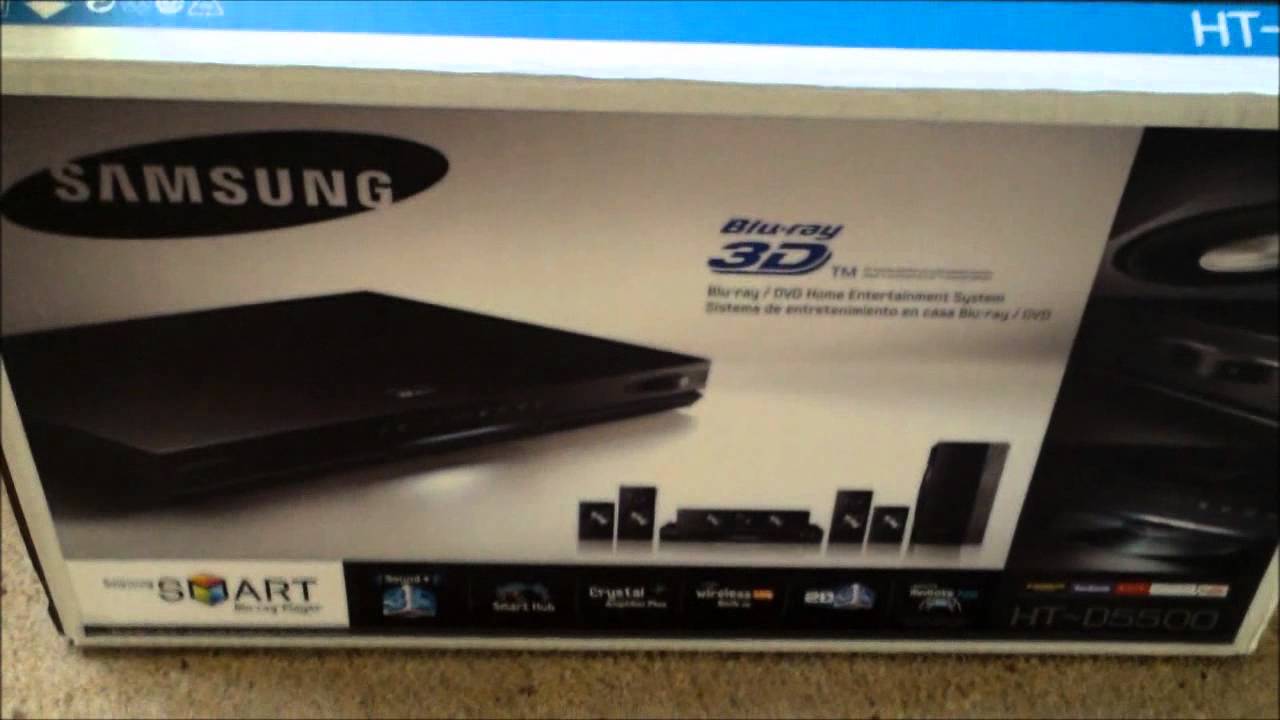This is a blurry image, likely taken with a smartphone, of a Samsung Blu-ray 3D DVD home entertainment system in its original packaging. The box, which appears to be placed on a light brown carpet, has a blue top with a white Samsung logo situated in a black oval in the upper left corner. To the right, the text reads "Blu-ray 3D" followed by "Blu-ray DVD home entertainment system." The box features a detailed illustration of the system, which includes a sleek, black Blu-ray player highlighted in the center-left, accompanied by five smaller speakers depicted in smaller detail below. The bottom section of the box includes some fine print and additional logos, among them "Samsung Smart" and the model number "HT-D5500." The overall color scheme is black, white, blue, gray, with touches of orange, yellow, and red. The photograph appears casual and unprofessional, possibly intended for an online marketplace listing.